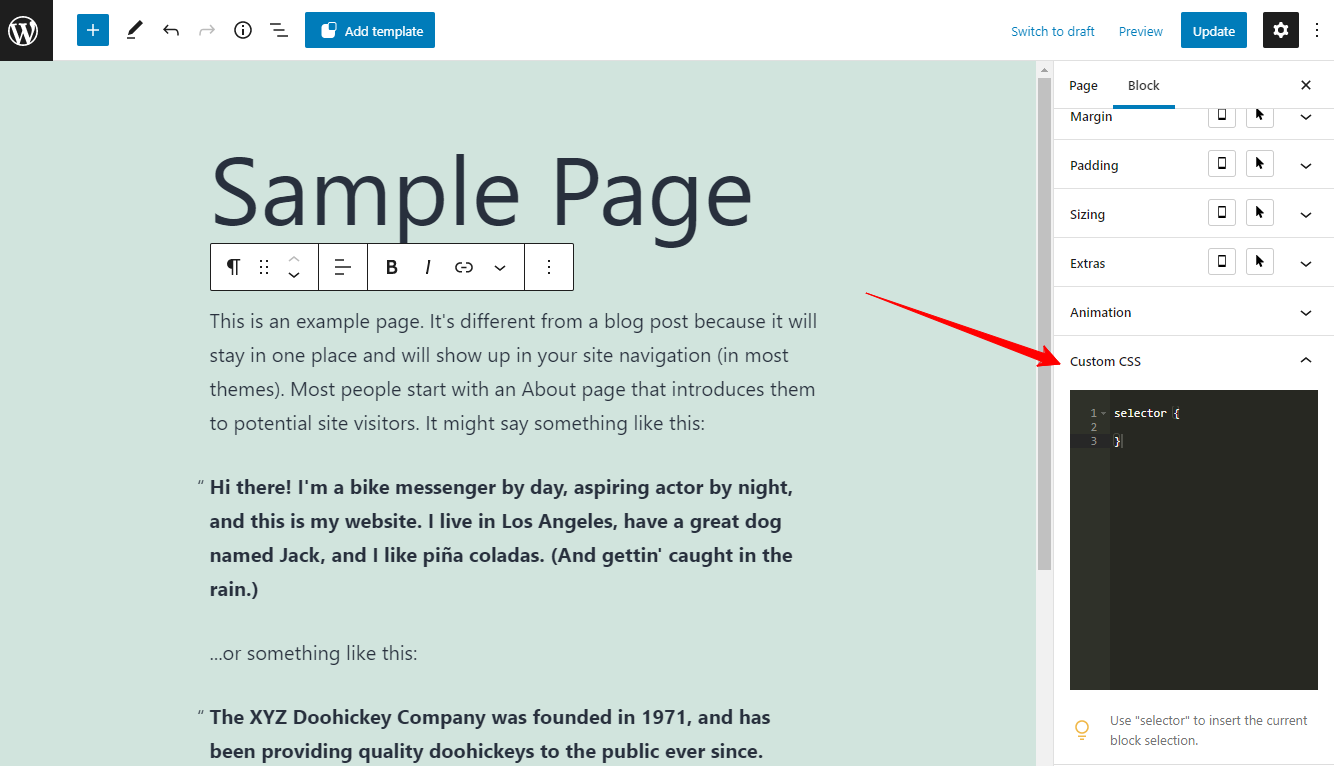The image depicts a WordPress interface in which a user is customizing a page template. In the top left corner, the WordPress logo is visible, confirming the platform being used. The central workspace displays a sample page labeled "Sample Page” with accompanying placeholder text: "This is an example page. It’s different from a blog post because it will stay in one place and will show up in your site navigation. Most people start with an About page that introduces them to potential site visitors." 

Around this content, a text editor widget is active, offering options to format text as italic or bold, indicating that the user is currently editing the text. On the right-hand side, a settings pane is open, which permits the adjustment of various page or block elements. Notably, a red arrow highlights a section titled "Custom CSS," suggesting that the user has the option to directly modify the page's underlying code by inputting custom CSS code in the designated area. This detailed setup illustrates the flexible and powerful customization tools available within WordPress for building and managing professional websites.